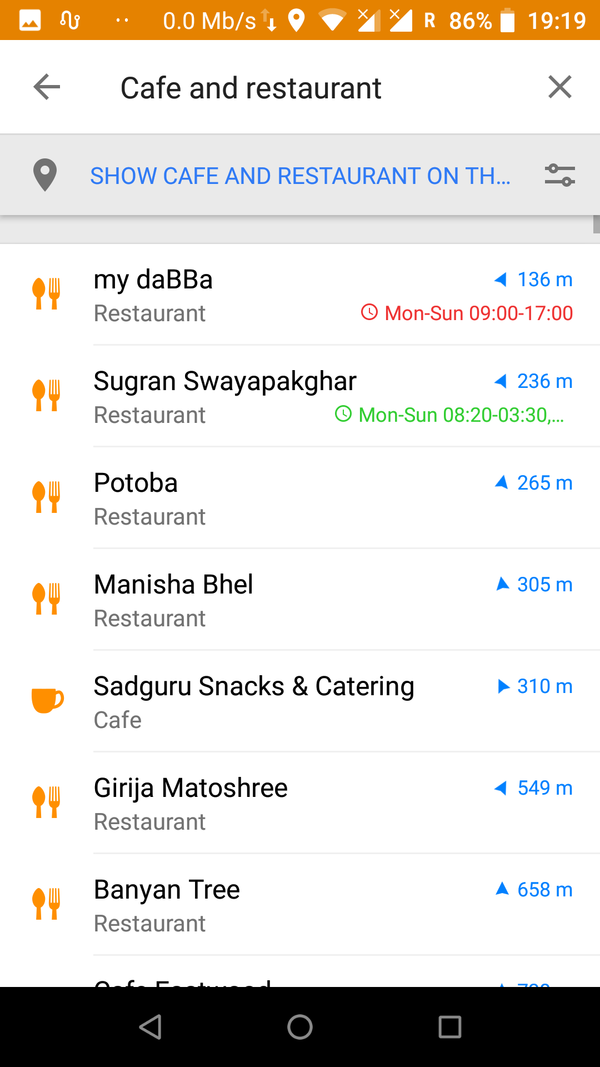**Screenshot from a Mobile Phone**

The top section of the screenshot displays an orange banner with a white graphic consisting of a square that includes some mountains at the bottom and an orange sky above. Adjacent to this, there is a small circle with a line that curves upwards and downwards, ending in a circle at the top, accompanied by two dots. Below this graphic, the text reads "0.0 Mbps" with an up arrow and a white down arrow, indicating network speed.

Adjacent to the data speed indicators, various icons are visible: a location icon, a WiFi signal indicator, a cell phone signal icon, a capital letter "R" with "86%" indicating network strength or battery state, and a battery icon showing 86% charge next to the current time, "19:19".

Below these indicators, there is a white banner featuring a left arrow on one end, the text "Cafe and Restaurant" in the center, and an "X" on the other end. This is followed by a gray banner that includes a location marker icon and the partially obscured text "Show cafe and restaurant on the...".

Descending further, a white background displays a series of icons and text. First, a spoon and fork icon is followed by "myDAPA," which is emphasized with uppercase letters "DAPA". Next, an identical icon represents "Sugar and Swayapak," spelled "S-U-G-R-A-N-S-W-A-Y-A-P-A-K-G-H-A-R". 

Following these is "Potoba" linked to "Manisha Bhel," both marked as restaurants, with "Manisha Bhel" spelled "M-A-N-I-S-H-A, B-H-E-L". Subsequent entries include a coffee mug icon symbolizing a cafe and the text "Sadgura Snacks and Catering".

Continuing with the list, a spoon and fork icon marks "Georgia Matosheri" ("G-I-R-I-G-A-A, M-A-T-O-S-H-R-E-E") and "Banyan Tree".